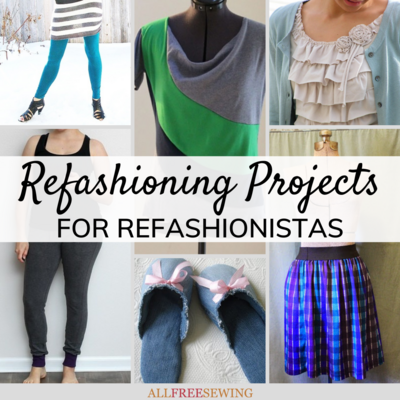The image, an advertisement for refashioning projects for refashionistas, is a collage featuring various fashion pieces, each contributing to a relaxed and loungewear style. Dominating the center, in italicized black letters, is the text "Refashioning Projects for Refashionistas," with "All Free Sewing" indicated at the very bottom.

In the upper left corner, there's a snowy background behind a woman showing only from the waist down, wearing a long gray and white striped shirt paired with aqua leggings and black high heels. Next to it, a mannequin showcases a gray shirt with a green banner across the chest. Further right, another image captures a woman from the neck to the waist, dressed in a light blue cardigan over a ruffled white blouse.

In the lower left corner, there's a woman, visible from the waist down, dressed in gray leggings with purple cuffs and a black tank top, standing against a beige wall above hardwood flooring. Centered below is an image of blue-gray slippers adorned with pink bows. Finally, the bottom right corner features a mannequin wearing a plaid blue skirt with a black waistband. The feminine and comfortable styling of the clothes suggests they are perfect for lounging or casual wear.